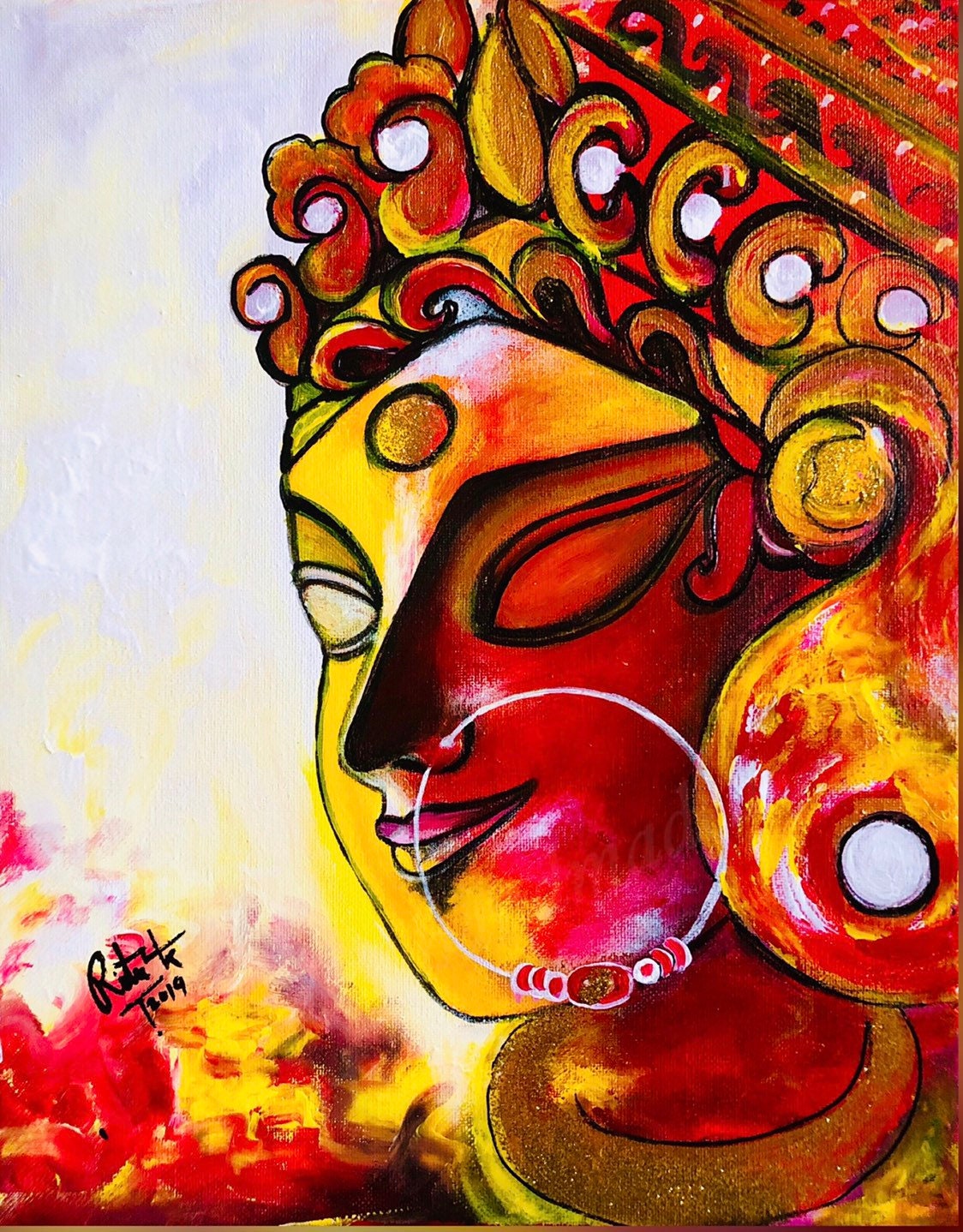The image appears to be a modern abstract watercolor painting, potentially using oil paint techniques, of an Asian woman or a Buddha-like figure. The painting prominently showcases a semi-profile view of the face, which gazes to the left from the viewer's perspective. The artwork features a bold color palette predominantly consisting of deep reds and yellows with touches of gold.

The face of the figure is divided into two distinct hues: the left side is yellow while the right side is red. The facial features include a slanted, nondescript eye outlined in black, and a sharply defined jawline and nose. A large white nose ring decorated with beads, including a central oval bead and three pink beads on each side, hangs from one nostril and extends down to the chin.

Adorning the top of the head is an intricate headdress with elaborate swirls and wave patterns, resembling gold and jeweled embroidery, with elements that might include cloth and feathers. The headdress design includes elongated, curvilinear motifs, potentially similar to fleur-de-lis. The right ear of the figure features a large white circle, adding to the detail.

The neck of the figure is painted predominantly in red and is encircled by a beautiful gold necklace or possibly a circular ornament. The background of the painting consists of shades of gray and yellow, transitioning to red and yellow towards the bottom.

In the bottom left corner of the image, there is the artist's signature, which appears to read "Rita TR" or "Roto 4k," along with the year "2019."